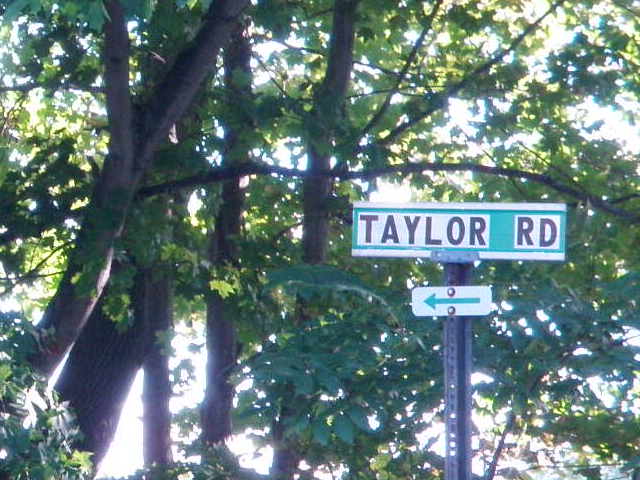The photograph captures an outdoor scene on a bright, sunny day, featuring a prominent green street sign reading "Taylor Road" in black text highlighted by a white background behind each letter. This rectangular sign is bordered by two white stripes at the top and bottom. Positioned below it, attached to the same dark gray, perforated steel pole with two bolts, is a smaller white sign with a green left-pointing arrow. In the background, the sky appears almost white due to the intense sunlight, and numerous tree trunks and branches stretch outward, adorned with a mix of green, light green, and yellow leaves that dapple in the sunlight.